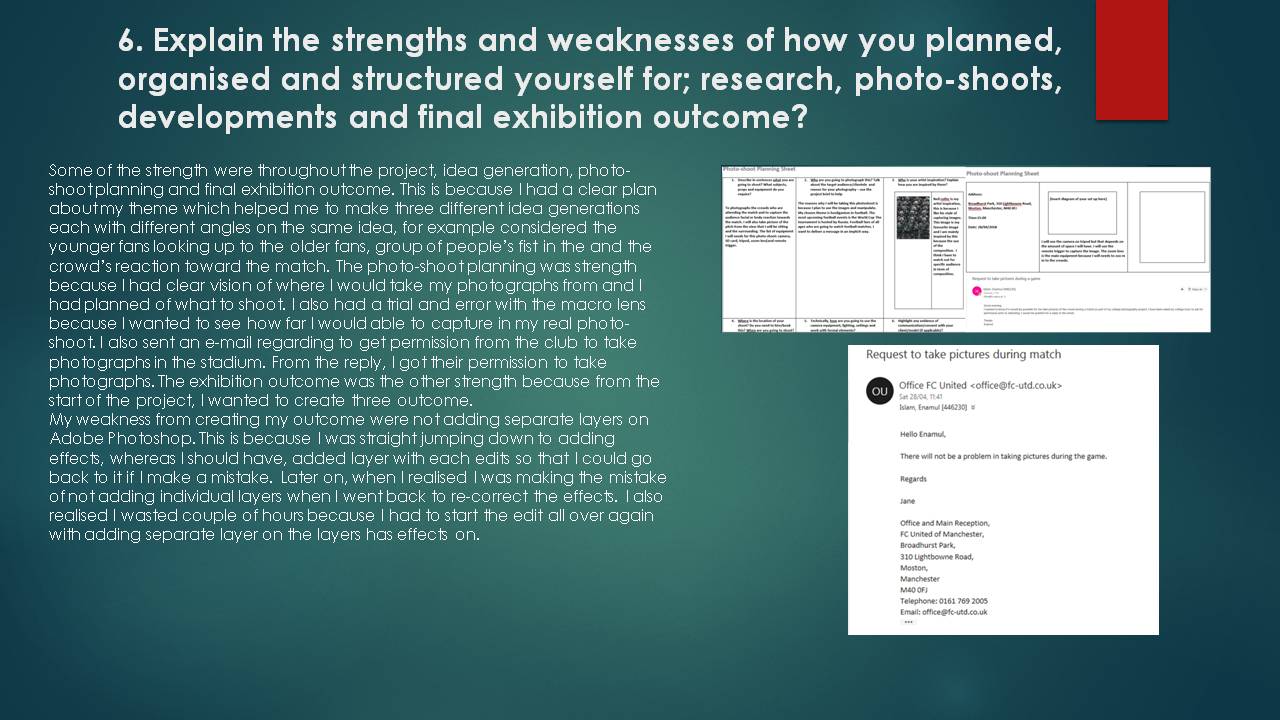This image depicts a detailed Q&A slide from a presentation, focusing specifically on question number 6. The background is a nuanced gradient, transitioning from light green in the center to dark green at the edges, with white text providing clarity against the backdrop. The question, prominently positioned in the top left corner, reads: "Explain the strengths and weaknesses of how you planned, organized, and structured yourself for research, photo shoots, developments, and final exhibition outcomes."

Below the question, a detailed response is elaborated in three smaller paragraphs, each discussing various aspects of the subject's planning and organizational skills. The answer outlines strengths such as a clear theme and well-executed idea generation, photo shoot planning, and final exhibition outcomes. Specific examples highlighted include strategic plans to capture different perspectives, such as the dynamics between younger fans and older fans, crowd reactions, and the intricacies of photographing matches.

On the right side of the slide, there are two white graphic boxes containing additional information. The top box is rectangular and horizontally aligned, while the lower box is more of a square shape. These boxes include charts and a dialogue between the presenter and an entity identified as "Office FC United," discussing permissions for taking pictures during a match. The overall presentation is rich in detail, effectively blending comprehensive written content with visual aids.